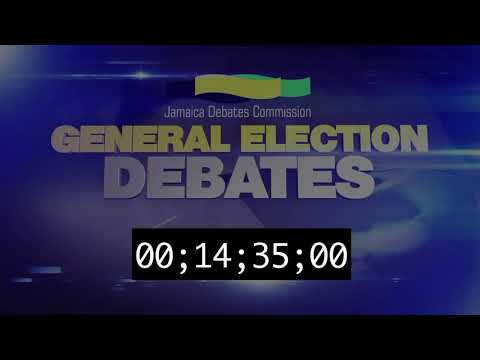The image is a detailed graphic with a text overlay presented against a striking blue background enhanced with various colored effects, including white lighting regions and ethereal orbs. The main text is organized into three lines: "Jamaica Debates Commission" in white, "General Election" in prominent yellow, and "Debates" in bold gray. Above this text, there are two wavy banners—one yellow and one mint green—reflecting the colors associated with Jamaica. At the bottom, a black rectangular box displays a timestamp with the numbers "00;14;35;00" in white text. The blue background is further accentuated with swirly yellow and green rectangles at the top and streaks of white lighting in the upper left and lower right corners.